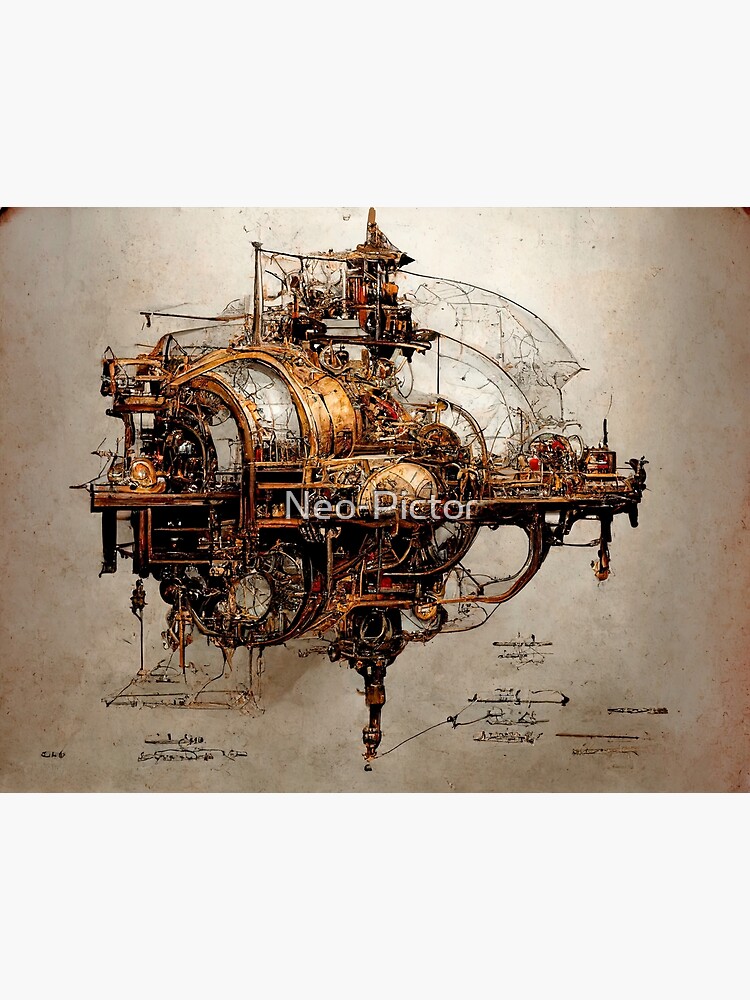The image is an intricate, steampunk-inspired drawing featuring a unique, orange-colored airship or floating contraption. The artwork is labeled with a watermark reading "Neopictor," N-E-O-P-I-C-T-O-R. The airship appears to be a conglomeration of gold, bronze, and some silver parts, including gears and possible globes, suggesting it could be a futuristic city or detailed plans for such a creation. The design showcases multiple openings on the sides and a mix of wood and metallic elements, including a drum-like portion with silver or gray highlights. There is also some barely legible writing at the bottom, adding to the antique and complex nature of the piece. Overall, the detailed portrayal combines old-fashioned aesthetics with a fantastical, mechanical theme, making the artwork both unique and intricately detailed.